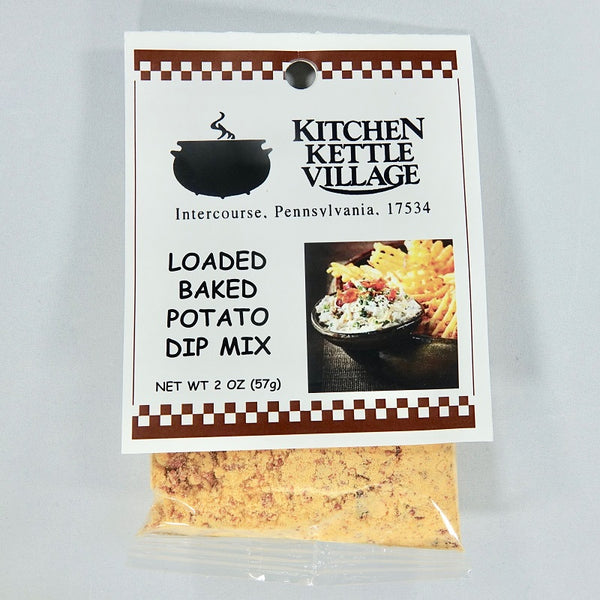This photograph showcases a product from Kitchen Kettle Village: a loaded baked potato dip mix. The dip mix is packaged in a clear plastic bag containing an orangish-yellow powder, possibly with reddish specks. The plastic bag is partially visible at the bottom, revealing a textural, granular substance inside.

Stapled to the top of the bag is a white cardboard label with intricate details. The label features maroon borders adorned with a triangle pattern, creating a distinctive frame at both the top and bottom. Prominently displayed at the top center is a silhouette of a pot with steam rising from it, accompanied by the text "Kitchen Kettle Village" in black letters. Below this, in a clear, orderly layout, the label indicates the location: "Intercourse, Pennsylvania, 17534." 

On the left side in Comic Sans font, it states "Loaded Baked Potato Dip Mix, Net WT 2 OZ, 57 grams." To the right is an image depicting a small bowl of creamy dip, flanked by a plate of crispy waffle fries, hinting at the end product. This detailed cardboard label serves both as an appealing visual and informative guide to the mix inside the plastic bag.